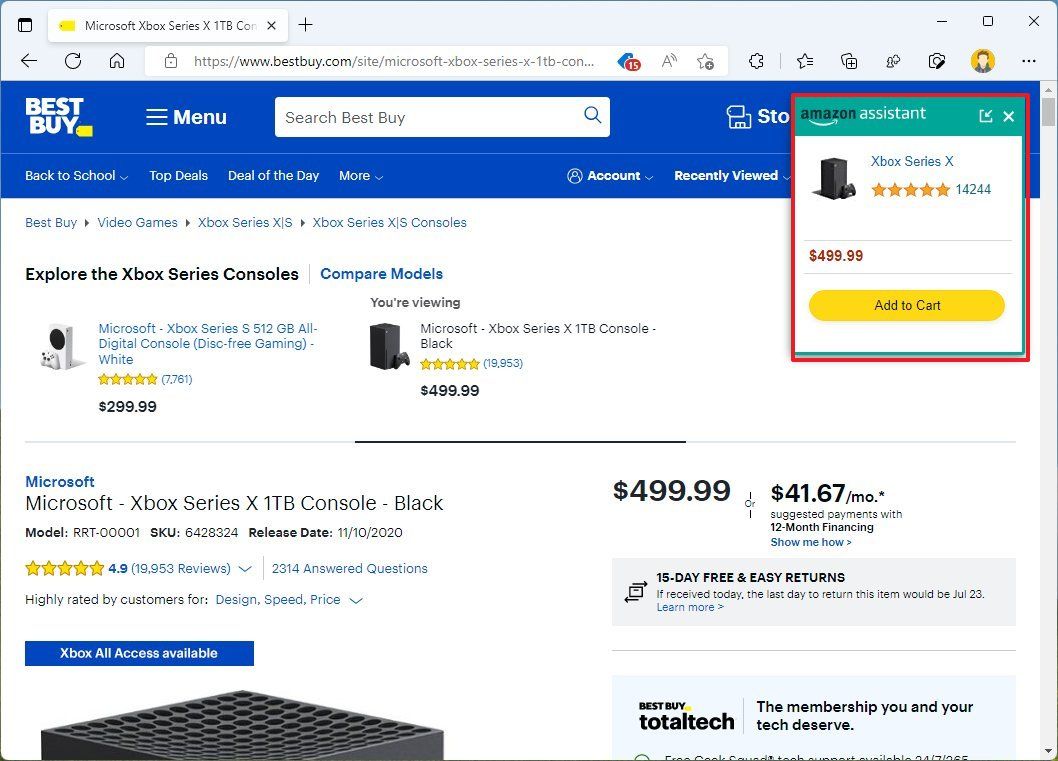The image showcases a product page on the Best Buy website. At the top, the signature Best Buy logo is displayed prominently within a yellow tag icon. Alongside it is a search box inviting users to "Search Best Buy." In the top corner, there's an Amazon Assistant feature highlighting a product with a red outline around it. The featured product is the Microsoft Xbox Series X 1TB Console in Black, released on November 10, 2020. The console has received a stellar 5-star rating and is priced at $499.99, with financing options available at $41.67 per month for 12 months. Best Buy also offers a 15-day return policy, meaning if purchased today, the return deadline would be July 23.

The product description includes the model number, SKU, and promotional messages regarding Best Buy’s Total Tech membership, emphasizing the support and benefits available to members. The displayed image of the Xbox Series X reveals its sleek black design, resembling a minimalist tower. The overall website design is predominantly white with Best Buy's signature bright blue accents, creating a clean and recognizable interface. The page provides various categories and options for browsing the website, reflecting Best Buy's extensive product range.